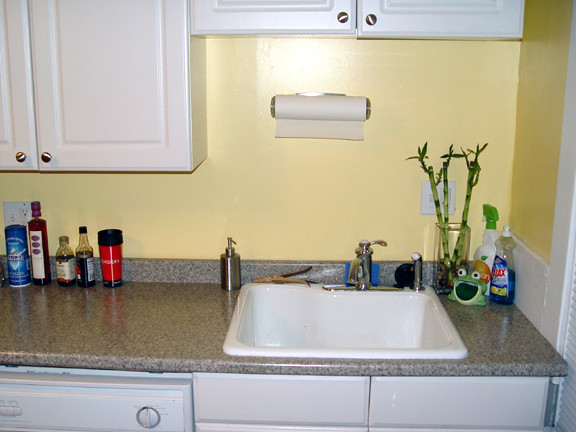This color photograph captures a well-maintained kitchen counter with a detailed array of items. The countertop itself is gray and appears to be made of granite or a similar stone. Above, the kitchen features white cabinets adorned with gold-colored knobs, complemented by a vibrant yellow wall that adds a warm touch to the scene. 

At the bottom left corner of the image, the upper part of a dishwasher is visible. Resting against the back of the counter, a variety of items are neatly organized. From left to right, there's a blue canister, followed by a tall red bottle, a small glass bottle, a slightly taller glass bottle, and a red travel coffee cup with a black lid.

Centrally located above the gray kitchen sink, a sleek silver paper towel holder dispenses a roll with the paper extending from behind. The sink itself boasts a pristine white porcelain basin, indicating it is empty. Positioned at the back left of the sink is a silver pump dispenser, likely containing hand soap. Attached on the right side of the sink is a dish sprayer for added utility.

To the right of the sink, a glass square-shaped vase holding three elegant bamboo stalks adds a touch of greenery. Adjacent to it, there’s a white spray bottle with a green nozzle, a half-full bottle of blue Ajax dishwashing liquid, and a charming small frog figurine with a wide mouth, cleverly holding a sponge inside. This thoughtfully arranged countertop is both functional and visually appealing.